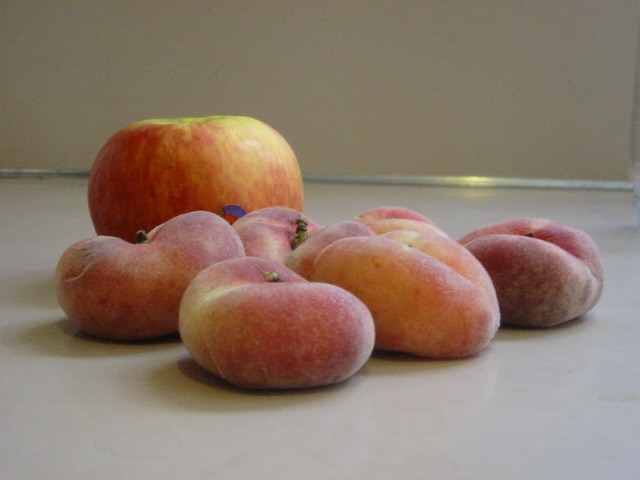This close-up photograph features an assortment of fruits displayed on a white surface, which could be a table or floor. The image is characterized by poor lighting that somewhat mutes the colors. The main subjects are a red and green apple positioned towards the back and several misshaped peaches in the foreground. The apple, which resembles a Honeycrisp, is primarily orange-red with light green stipples, particularly near the stem, creating a variegated appearance. The peaches, numbering between four and six, exhibit a peculiar flattened form, as if they have been squished. They are fuzzy with a mottled coloration that transitions from deep, almost blackish red to lighter shades of yellow and green. These peaches also appear somewhat dried or aged, giving them an unusual, almost jelly bean-like shape. The setup suggests a casual, perhaps experimental arrangement of fruit.